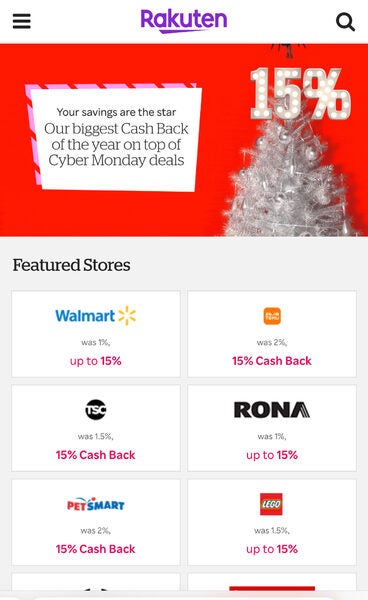The image displays a Rakuten website or application interface. At the very top, there is a white banner featuring the word "Rakuten" in purple text, partially underlined by a purple line that covers the letters A, K, U, and T. On the left side of this banner, a hamburger icon represented by three horizontal lines indicates the presence of a menu. On the right side, there is an eyeglass icon to facilitate searches.

Beneath the banner, a prominent red box highlights a 15% discount, adorned with a stylized white Christmas tree. Within this red box, a smaller white box contains the text "Your savings are the star. Our biggest cash back of the year on top of Cyber Monday deals."

Below the red box, the section titled "Featured Stores" showcases panels of various retailers offering significant cash back deals. The featured stores include:

- **Walmart**: Up to 15% cash back
- **Timu**: 15% cash back (visibility is somewhat unclear)
- **TSC**: 15% cash back
- **Rona**: Up to 15% cash back
- **PetSmart**: 15% cash back
- **LEGO**: Up to 15% cash back

Additional store panels appear to be present below but are cut off at the bottom of the image. This interface illustrates Rakuten's platform for accessing discounts and cash back deals from various retailers.